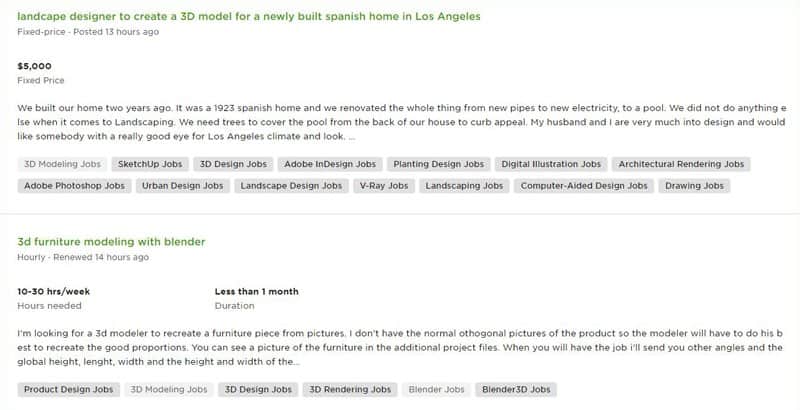This image features an advertisement page for 3D modeling services with a clean white background. 

In the top section on the left, there is green text offering a position for a "Landscape Designer to create a 3D model for a newly built Spanish home in Los Angeles." The job is listed as a fixed-price project, posted 13 hours ago, with a budget of $5,000. Below this, there are details about the home and relevant tags.

The second section of the advertisement lists a job titled "3D Furniture Modeling with Blender." This is an hourly position, renewed 14 hours ago, with an estimated commitment of 10 to 30 hours per week. The project duration is expected to be less than one month. Similar to the first listing, this section also includes additional information and tags.